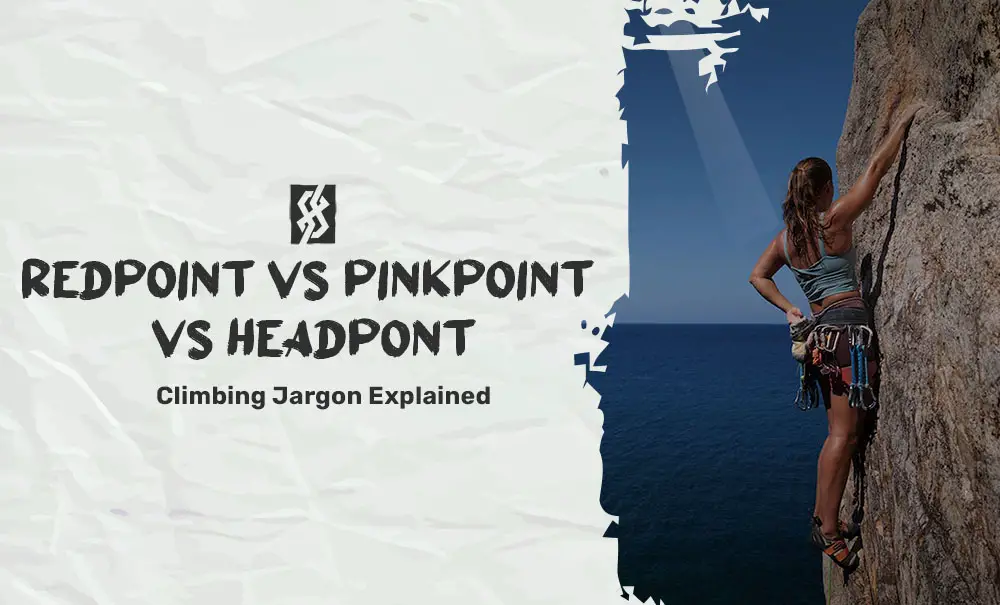This potential book cover features a split design with the left half dominated by a clean, white background. The title "Red Point vs. Pink Point vs. Head Point" is prominently displayed in bold black text, with the subheading "Climbing Jargon Explained" in smaller black text beneath it. 

The right half showcases a striking photograph of a woman in the midst of an intense climbing session on a large, dark gray rock formation. She is dressed in a blue tank top and blue denim shorts, equipped with a climbing belt adorned with various tools and gear. Her right hand clutches a rocky protrusion, while her left hand rests on her hip. She stands poised against the rock with her black climbing shoes that feature orange stripes. 

Above her, the scene is framed by a clear, blue sky, and below, a vast, blue body of water stretches out, emphasizing the height and daring nature of her climb. The composition effectively conveys the challenging nature of climbing, with the powerful imagery of the woman contrasted against the technical terminology of the title.